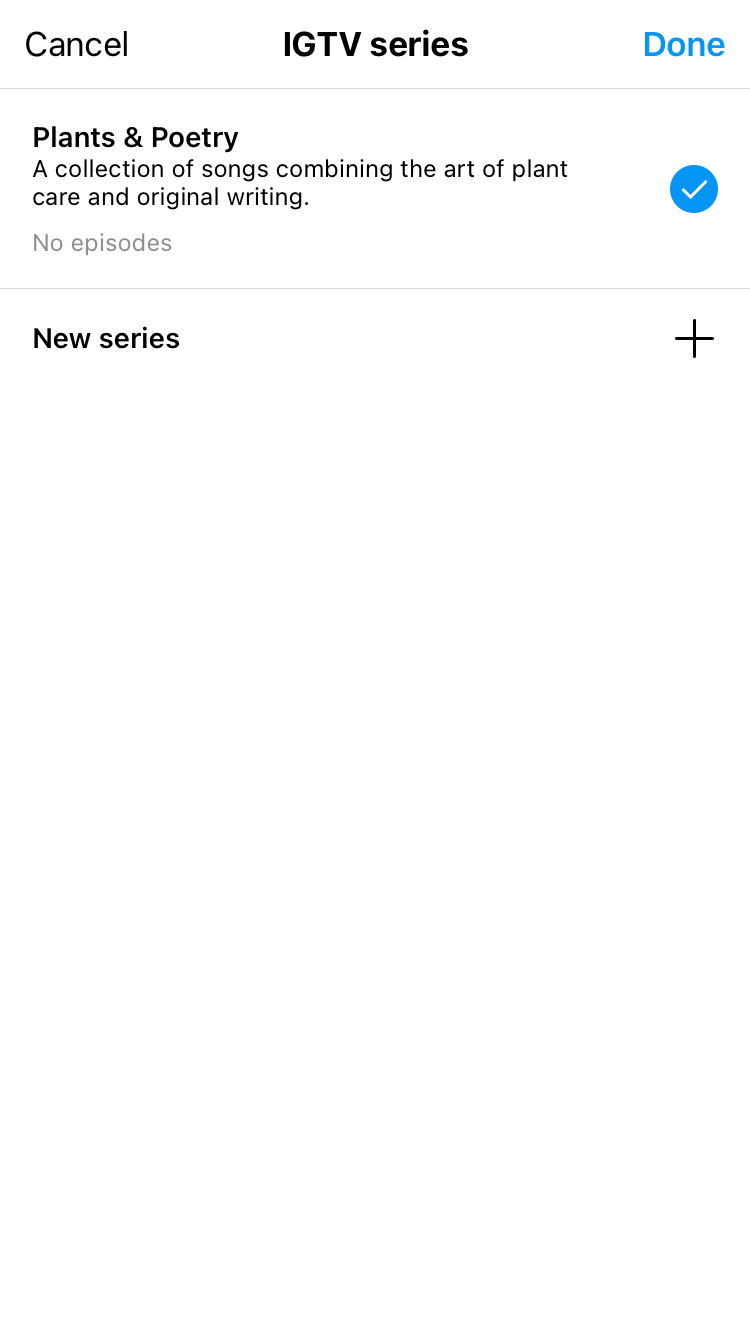Here's a detailed and cleaned-up descriptive caption for the image:

---

The image is a screenshot of a website with a completely white background. In the top-left corner, the word "Cancel" is visible in black letters. To the right of "Cancel," there is a white space, followed by the text "IGTV Series" in lowercase letters, and then another white space. To the far right of this, the word "Done" is displayed in blue letters. 

Directly below the word "Cancel," a gray line extends across the width of the screenshot. Below the gray line, the text "Plants and Pottery: A collection of songs combining the art of plant care and original writing" is clearly visible, with a white space to its right. To the further right of this space, there is a blue circle containing a white check mark, with the long part of the check mark pointing toward the right.

Beneath the descriptive text on the left, the phrase "No episodes" is written in gray letters. Another gray line is located below this text. Underneath this second gray line, "New Series" appears in bold black letters. Adjacent to this, there is a large white space, and positioned to the far right at the bottom of the screenshot is a black plus symbol made up of two intersecting lines forming a cross.

---

Let me know if you need any further adjustments!